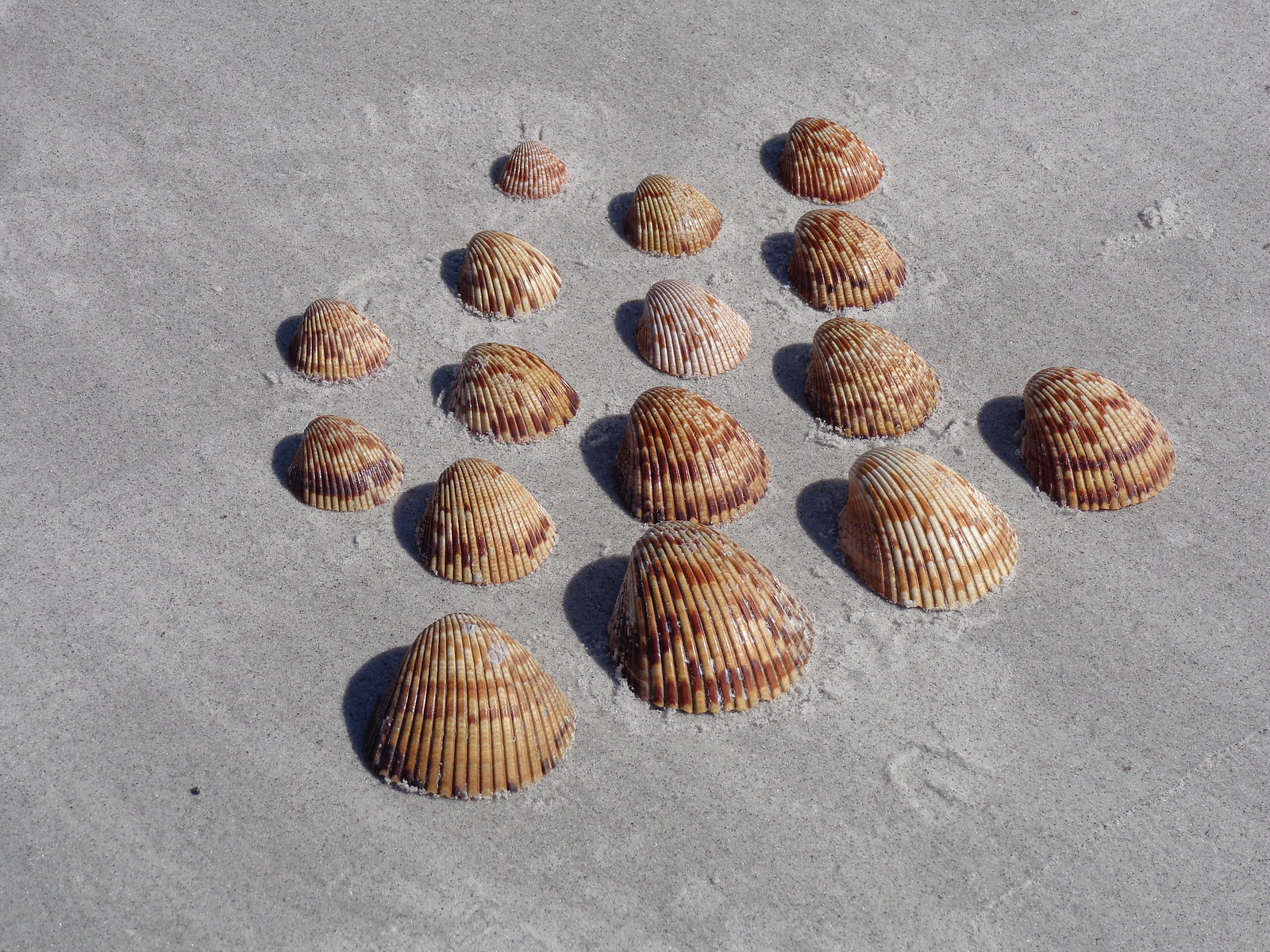The photograph showcases 16 seashells meticulously arranged in rows upon a fine, light gray sand. These shells, appearing to be scallop-like, are laid face down and face the same direction, indicating deliberate placement by a person. The shells are organized from bottom to top in a sequence: four in the first row, three in the second, four in the third, four in the fourth, and one on the fifth row. Each shell boasts a unique color pattern, featuring shades of dark brown, regular brown, light tan, and white, with distinctive vertical lines. Small shadows extend slightly in front of them, adding to the image's intricate detail. The sand's refined texture and subtle shading provide a tranquil backdrop for this orderly shell display.